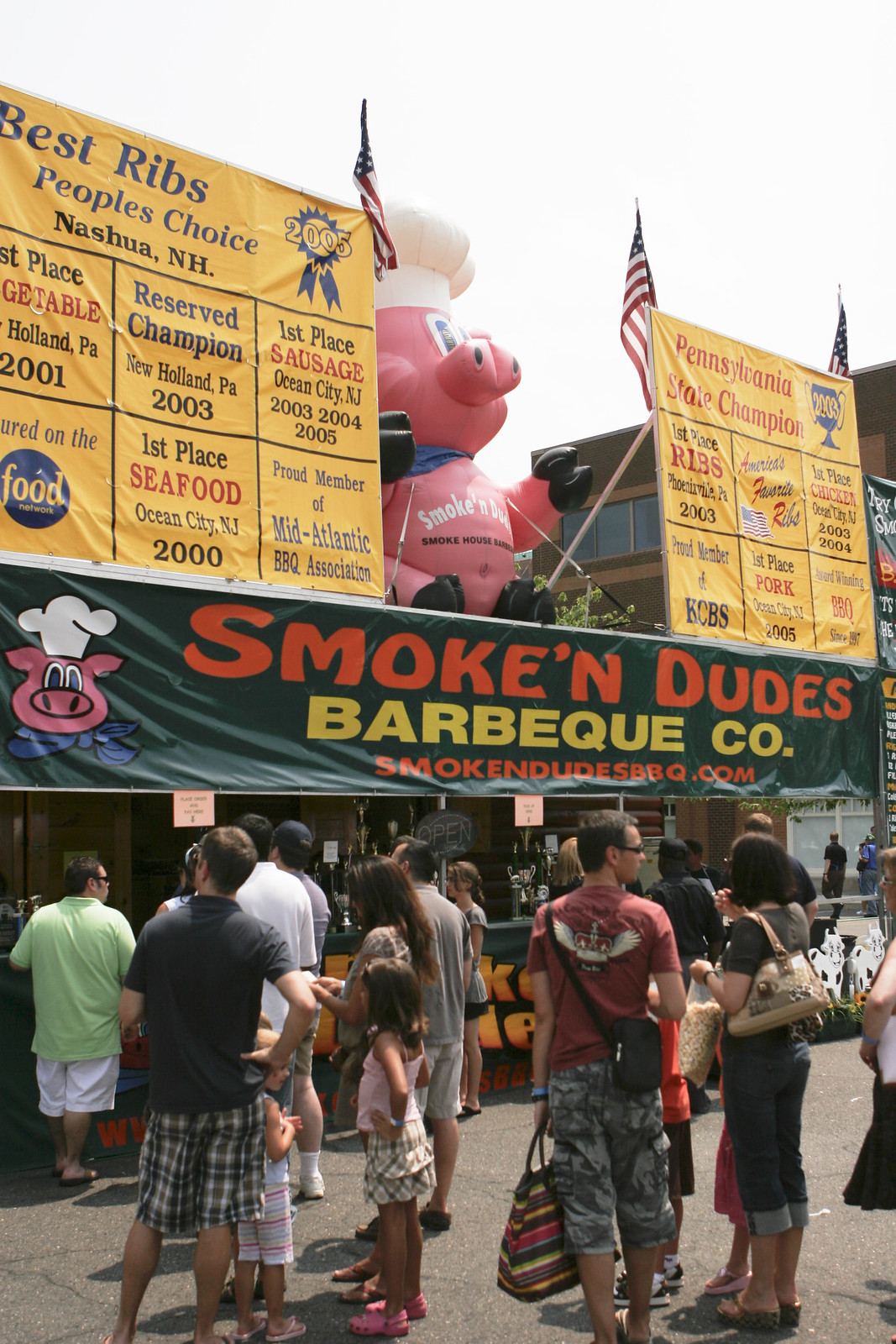This vertical rectangular photograph captures a vibrant scene at a state fair or carnival, centered on a bustling barbecue stand named "Smokin' Dudes Barbecue Company." The temporary, booth-like structure is adorned with a large green banner featuring the establishment's name in bold orange and yellow letters. Dominating the top of the booth is a large inflatable pink pig, donning a white chef's hat and a blue bowtie, flanked by two American flags. Below the banner, a sea of fairgoers clad in warm-weather attire, such as shorts and t-shirts, is seen eagerly standing in line to order food.

The pig stands as the booth’s quirky mascot, matched by a smaller version of its logo hanging from the main sign, amplifying the festive atmosphere. Surrounding the inflatable centerpiece are two yellow signs boasting the restaurant's impressive accolades: "First Place Seafood, Ocean City, New Jersey," "First Place Sausage, Ocean City, New Jersey," "First Place Ribs, Phoenixville, Pennsylvania," "First Place Pork, Ocean City, New Jersey," and titles like "Best Ribs, People's Choice" and "Pennsylvania State Champions." These awards underscore the enticing cuisine that Smokin' Dudes prides itself on, promising a savory experience for its patrons.